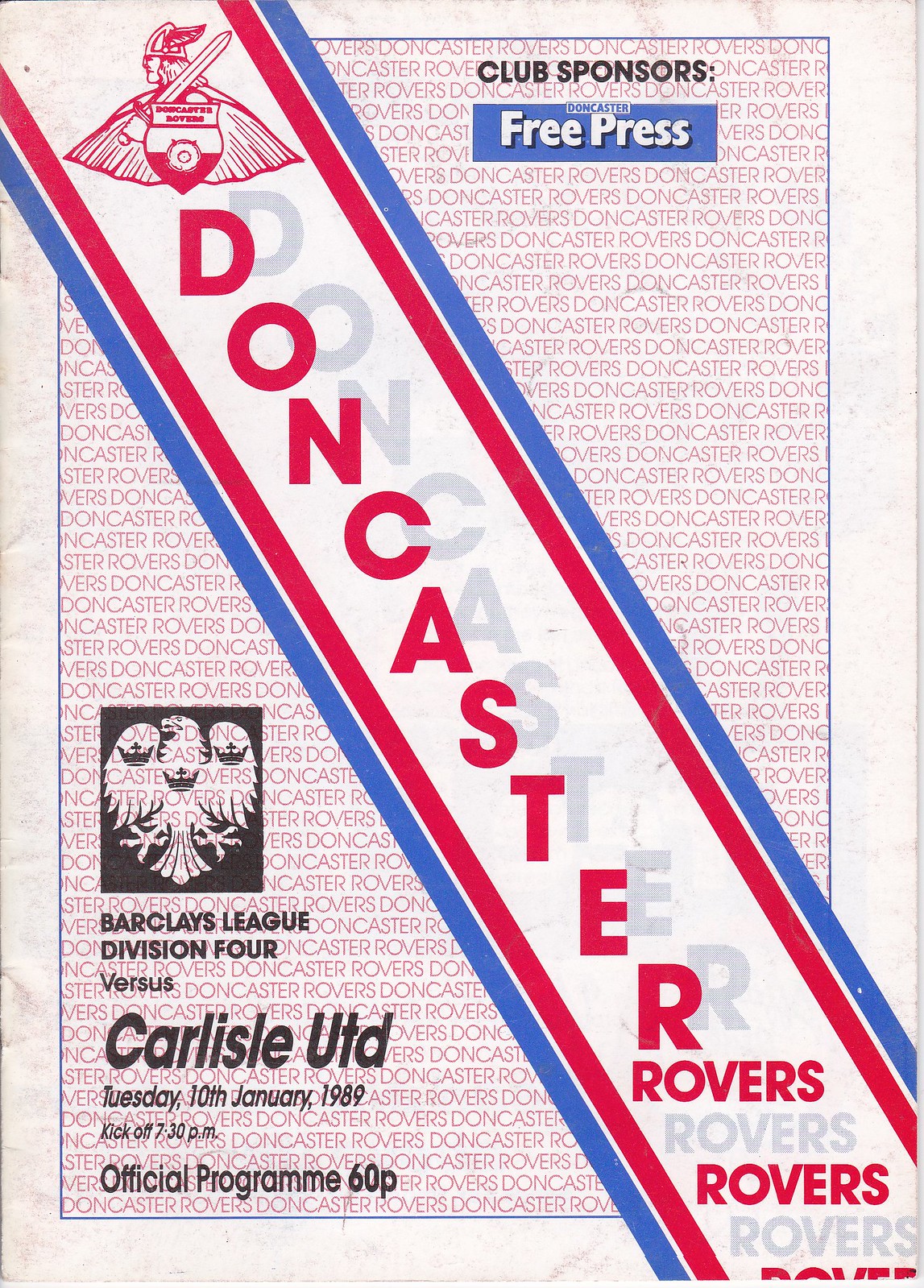This image is a photocopy of an old sports program cover for a soccer match, advertising a game between Doncaster Rovers and Carlisle United from the 1980s. The cover prominently features red and blue stripes along with red text repeatedly displaying "Doncaster Rovers." A ribbon, also reading "Doncaster Rovers," is interlayed across the design. It has white margins separated by a blue line. In the upper right-hand corner, a notation indicates "Club Sponsors Free Press." The left-hand side of the cover features detailed event information in black text: "Barclays League Division IV vs. Carlisle UTD, Tuesday, 10th January 1989, kickoff 7.30 PM," along with the price, “official program, 60p.” Additionally, an eagle symbol is located on the left-hand side of the image, contributing to the sports theme.